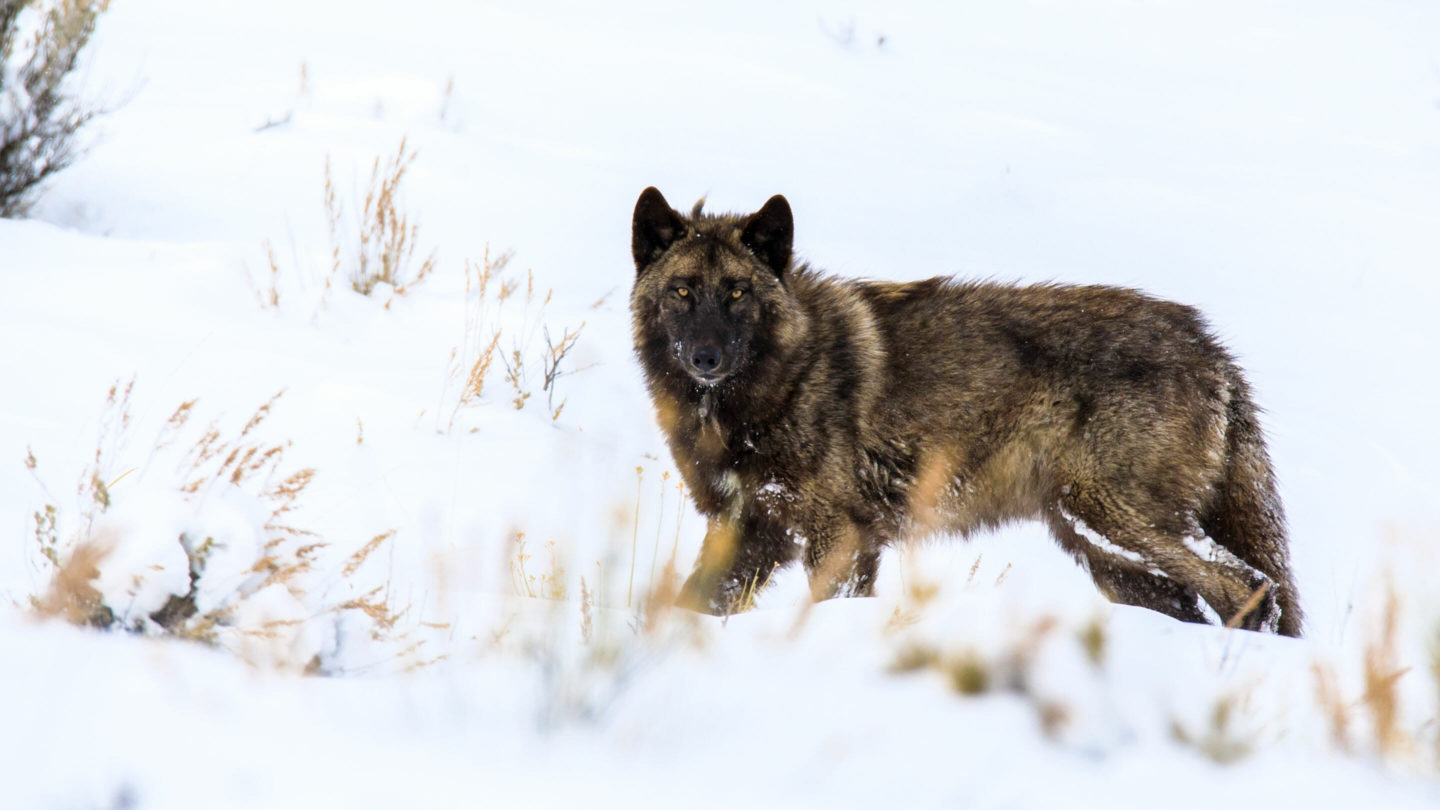Set against a picturesque winter backdrop, this photograph captures a striking dark grey and black wolf in a snowy, woodland setting. The wolf, standing in profile but with its head turned to gaze directly at the camera, boasts piercing deep yellow, almost orange eyes. The creature's dense fur shows hints of a light tan undercoat, contrasting with the darker tones of its ears, face, and chest, adorned with subtle black lowlights along its flanks. Amidst the foreground, which is slightly out of focus, a scattering of brown branches and dried grass protrude through the snow. The wintry forest around it is almost pure blue and white, deeply out of focus, which enhances the wolf's presence as the main focal point of the image. The serene daytime scene encapsulates the raw beauty of nature and the majestic demeanor of the wolf mid-stride through its snowy domain.